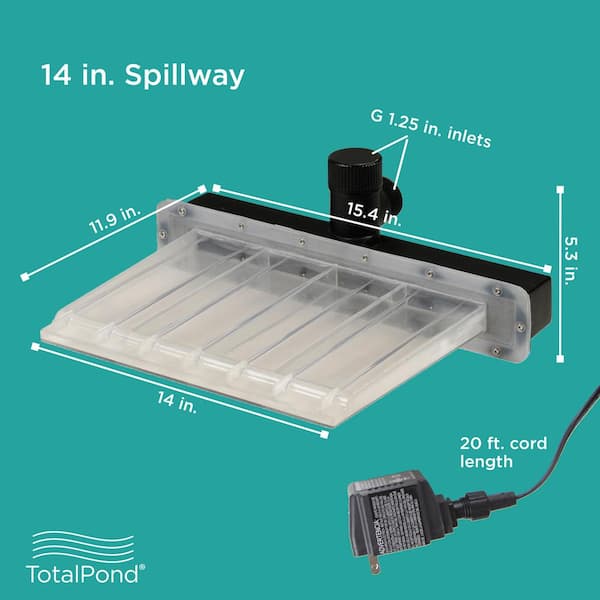The image illustrates a detailed diagram of a 14-inch spillway, designed for creating water features or ponds, prominently branded by Total Pond, with a trademark symbol above the "D." The scene is set against a solid teal background that encompasses the majority of the picture. The central focus is on the spillway device, comprising a clear plastic tray mounted on a black backing. The upper left-hand corner of the image displays the label "14 in. Spillway" in bold text. The spillway features several inlets, one of which appears suitable for attaching a garden hose, indicated by dimensions marked around various parts of the device—11.9 inches from back to front and 15.4 inches for the adjustable black part. On the bottom left corner, Total Pond's brand name and four wavy white lines stand out. In the bottom right corner, a 20-foot black cord with a plug is shown, ready to power the spillway.